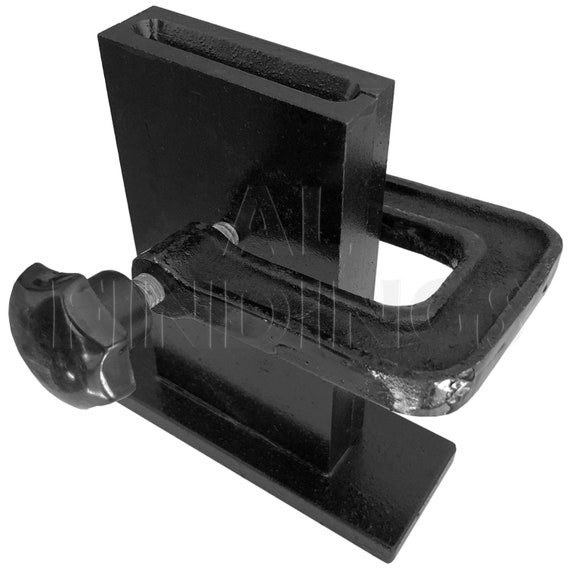In this detailed image, we see a black, U-shaped mechanical vise made primarily of metal, positioned on a shiny, black rectangular base. This vise features a threaded screw mechanism with a black plastic knob on the left side, which is used to tighten its grip around an object. The object in question appears to be a rectangular metal piece that is hollow in the middle and secured tightly within the vise’s grasp. The overall structure exudes a heavy-duty, polished finish, indicating possible recent painting or maintenance. Moreover, the image contains a faint watermark showing partial text, with discernible letters such as "AL" towards the top and fragments like "N, D, I, N, G, S" near the bottom, hinting at possibly the word "FINDINGS."